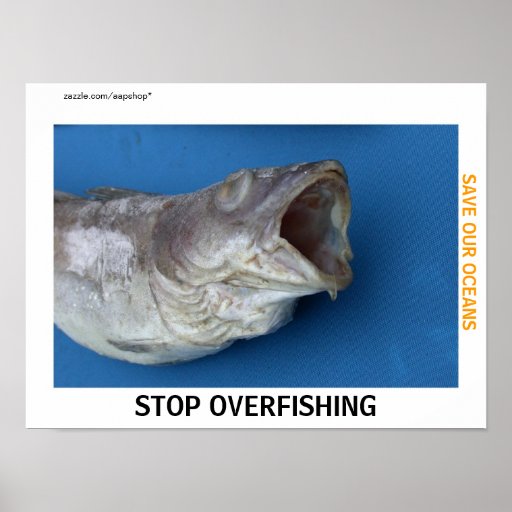The image is a poster featuring a photograph of a distressed or dead fish with its mouth gaping open, silvery-gray in color with dehydrated gills and gray eyes. The fish is set against a blue background, which is surrounded by a white border. On the white border, at the bottom in bold black uppercase letters, it says "STOP OVERFISHING." Along the right side of the border, written vertically in smaller yellow capital letters, is the message "SAVE OUR OCEANS." In the upper left-hand corner of the border, in lowercase black letters, appears the credit "zazzle.com/AAP shop*." This entire rectangular composition is placed within a gray gradient square that transitions from pale gray on the left to darker gray on the right. No other objects, texts, or people are visible in the image.